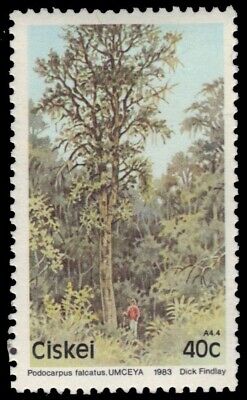This image features a low-resolution, blurry close-up of a postage stamp from Ciskei, characterized by perforated edges typically found on tear-apart stamps. The stamp, part of a collection mounted on a black background, illustrates a stylized forest scene with a central tall tree adorned with thin branches and foliage. Surrounding the tree are abstracted, stylized bushes and trees set against a pale turquoise sky. At the base of the tree stands a figure in a red shirt and white pants. The bottom left of the illustration reads "CISKEI," while the bottom right is marked "40C." Below the illustration, the white border includes the text "PODOCARPUS FALCATUS U-M-C-E-Y-A 1983 DICK FINDLAY."